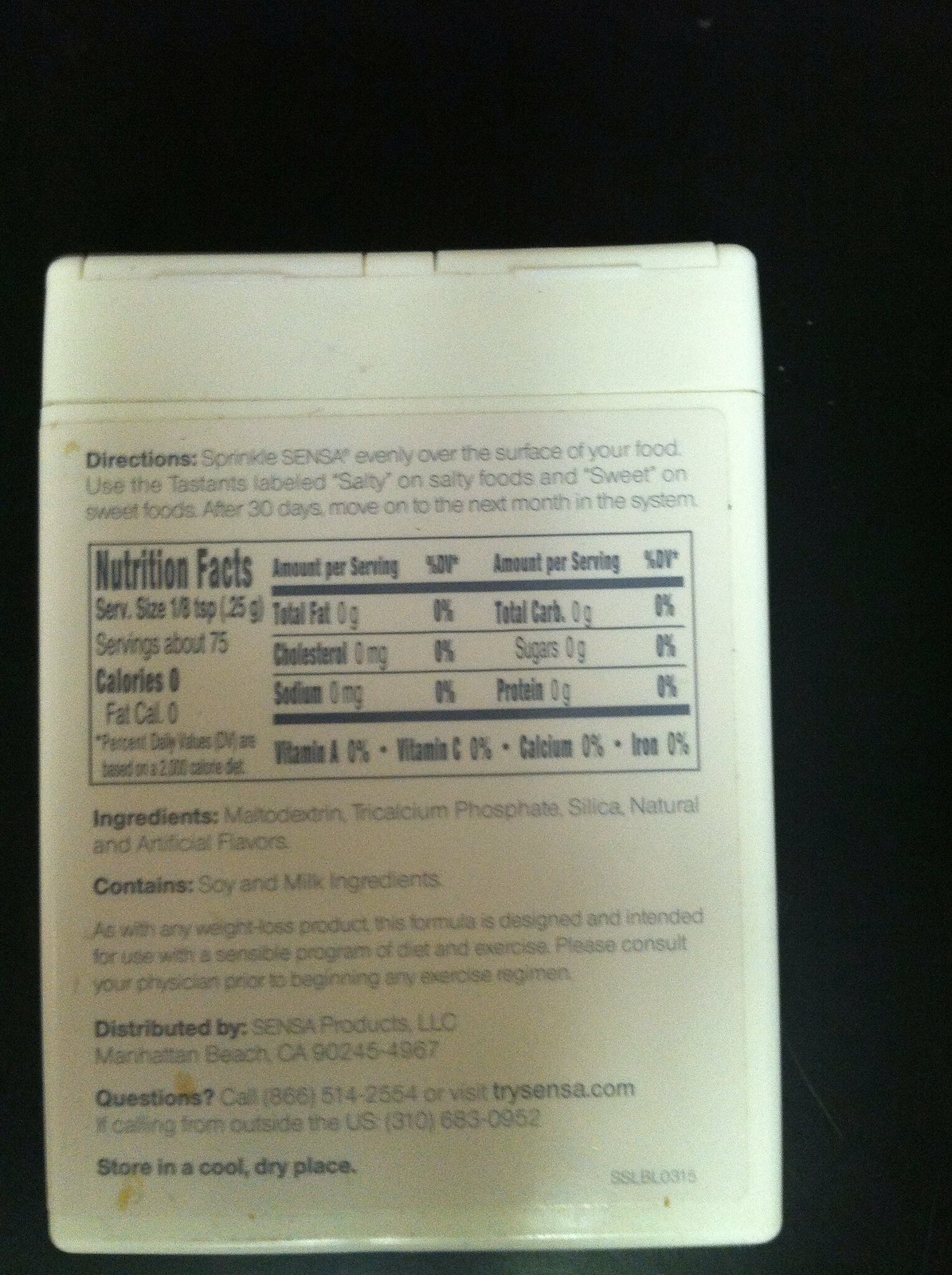The image showcases the nutritional facts and usage directions for a weight loss product in a white box set against a black background. The instructions advise users to sprinkle Sensa evenly over their food, using the tastants labeled 'Salty' for savory foods and 'Sweet' for sweet items. After 30 days, users should progress to the next month in the system. 

The nutritional information and a list of ingredients are provided, which include maltodextrin, tricalcium phosphate, silica, and both natural and artificial flavors. The product contains soy and milk ingredients and is described as a sugar and salt substitute. A note emphasizes that the product is intended to be used alongside a sensible diet and exercise program, and advises consulting a physician before starting any exercise regimen. 

The product is distributed by Sensa Products based in Manhattan Beach and their website trisensa.com is provided for more information. At the bottom, there's a storage instruction to keep the product in a cool, dry place.